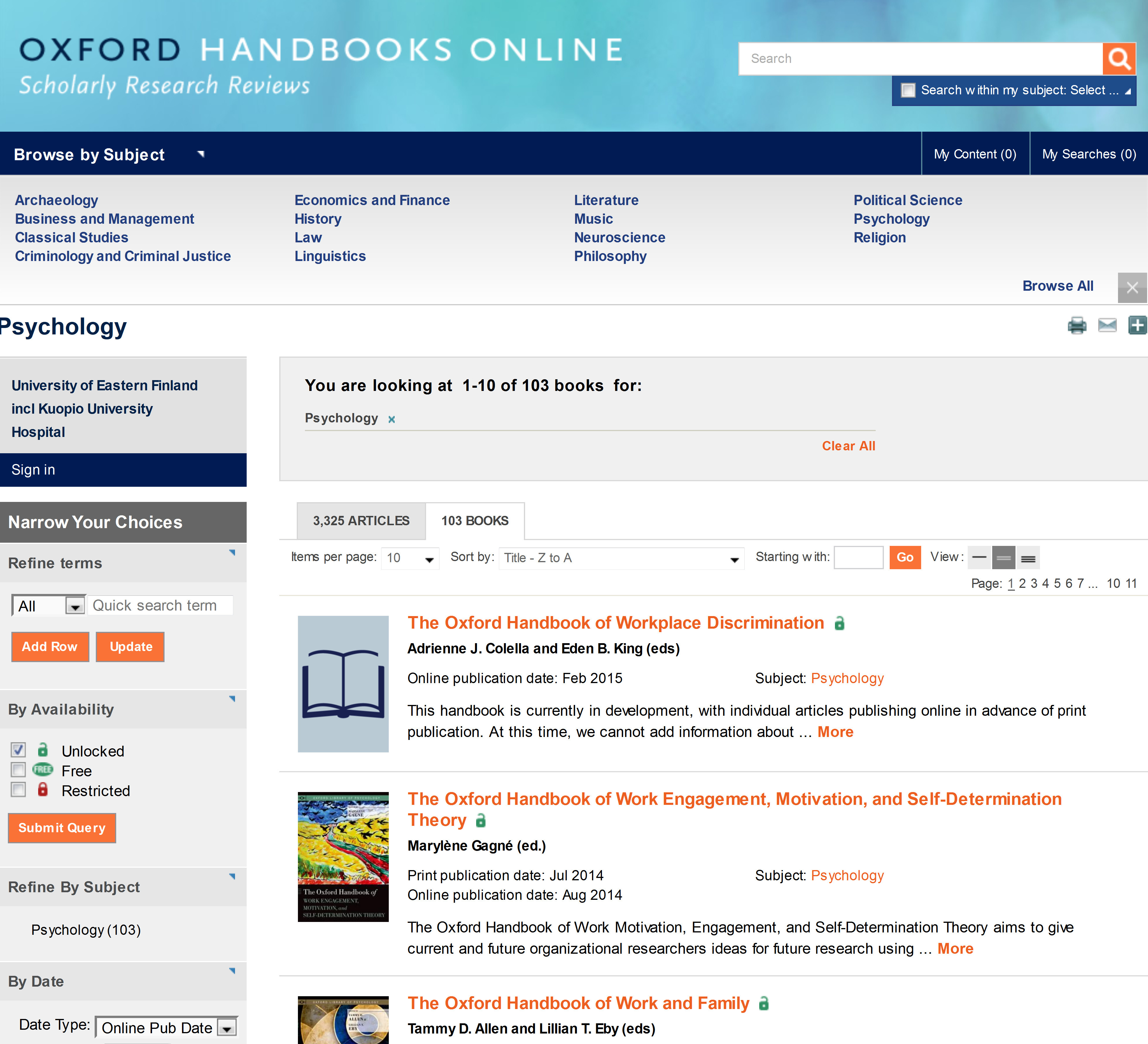The website for Oxford Handbooks Online is displayed with a light blue banner at the top, featuring the word "Oxford" in navy blue, followed by "Handbooks Online" in white letters, and underneath, "Scholarly Research Reviews" in italic white text. On the right side of the banner is a search bar accompanied by an orange search button symbolizing the Enter function. 

Beneath the banner, users can browse a variety of subjects which are organized into four columns. The subjects include Archaeology, Business and Management, Classical Studies, Criminology and Criminal Justice, Economics and Finance, History, Law, Linguistics, Literature, Music, Neuroscience, Philosophy, Political Science, Psychology, and Religion. The first four columns contain up to four subjects each, whereas the last column contains three subjects.

The opened page specifically displays psychology options. There is a search box to narrow down choices and refine search terms by availability, subject, and date. As a result of a search query, there are 103 book results shown, with a screenshot displaying the first few. 

The first book listed is "The Oxford Handbook of Workplace Discrimination." The title is in orange font, the authors' names are in black font, and the online publication date and subject are noted. There are also two lines summarizing the book.

The second book is titled "The Oxford Handbook of Work Engagement, Motivation, and Self-Determination Theory," followed by the "Oxford Handbook of Work and Family" as the third book in the list.